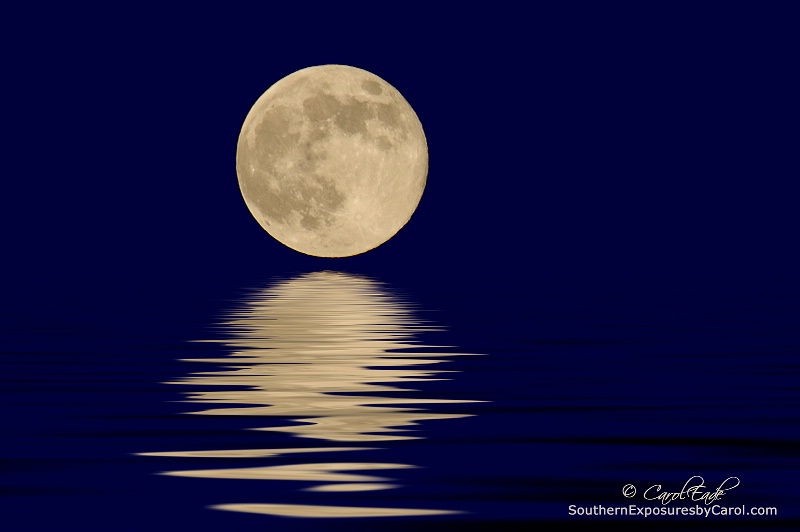The image is a rectangular artistic photograph featuring a full moon in a dark blue nighttime sky. The moon is situated nearly in the center toward the upper portion of the picture, showcasing distinct yellow and brown spots. The sky transitions smoothly from a solid dark blue to the slightly lighter hues near the horizon, devoid of any clear differentiation between the sky and the dark blue water below. Gentle ripples traverse the water surface, suggesting a serene lake or ocean under the moonlight. The moonlight casts a vivid reflection on the water, creating an ethereal glow. In the lower right-hand corner, small white text reads "Southern Exposures by carole.com," with a signature in yellow script just above it, appearing to be "Carole Eagle" though slightly unclear. The color palette comprises mainly of dark blues, white, light tan, and black, capturing the quiet, reflective beauty of an outdoor, nighttime scene.